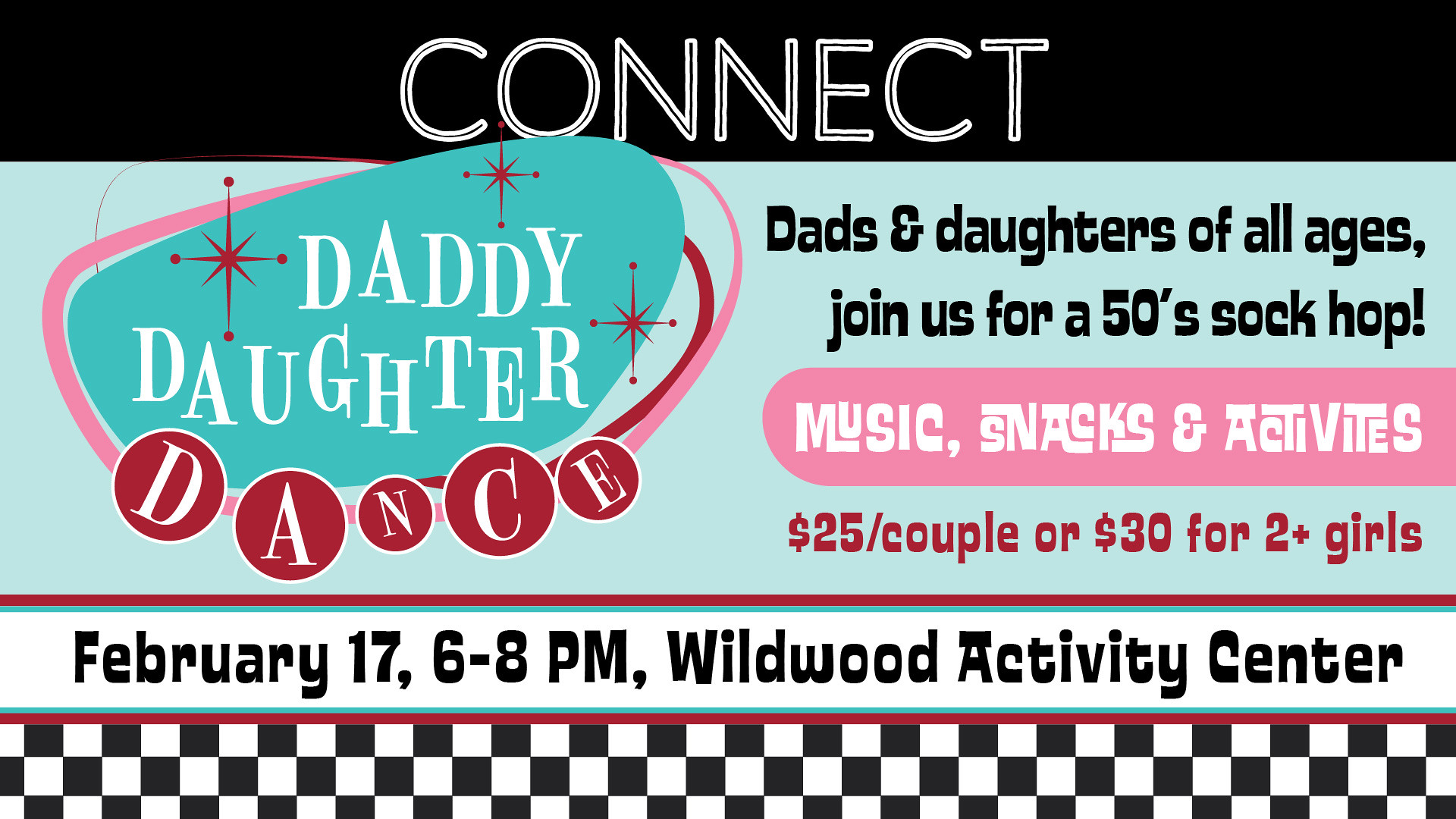This is a detailed color photo of an advertisement for a 1950s-style Daddy-Daughter Dance. The background is pale blue, and across the top is a black bar with the word "CONNECT" in white letters. Below the bar, there is a turquoise, kidney-shaped area outlined first by a pink line and then a red line. Inside this shape, in white text, it reads "Daddy-Daughter," accompanied by three red stars. Below this, in large red circles, the word "DANCE" is prominently displayed. 

The main text announces: "Dads and daughters of all ages, join us for a 50s sock hop!" Details about the event follow, stating: "Music, snacks, and activities. $25 per couple or $30 for two plus girls." At the bottom, there’s a black and white checkered banner giving it a distinct 1950s vibe. Below the main text, further details include: "February 17th, 6 to 8 p.m., Wildwood Activity Center." The words "music, snacks, and activities" appear again in white on a pink background.